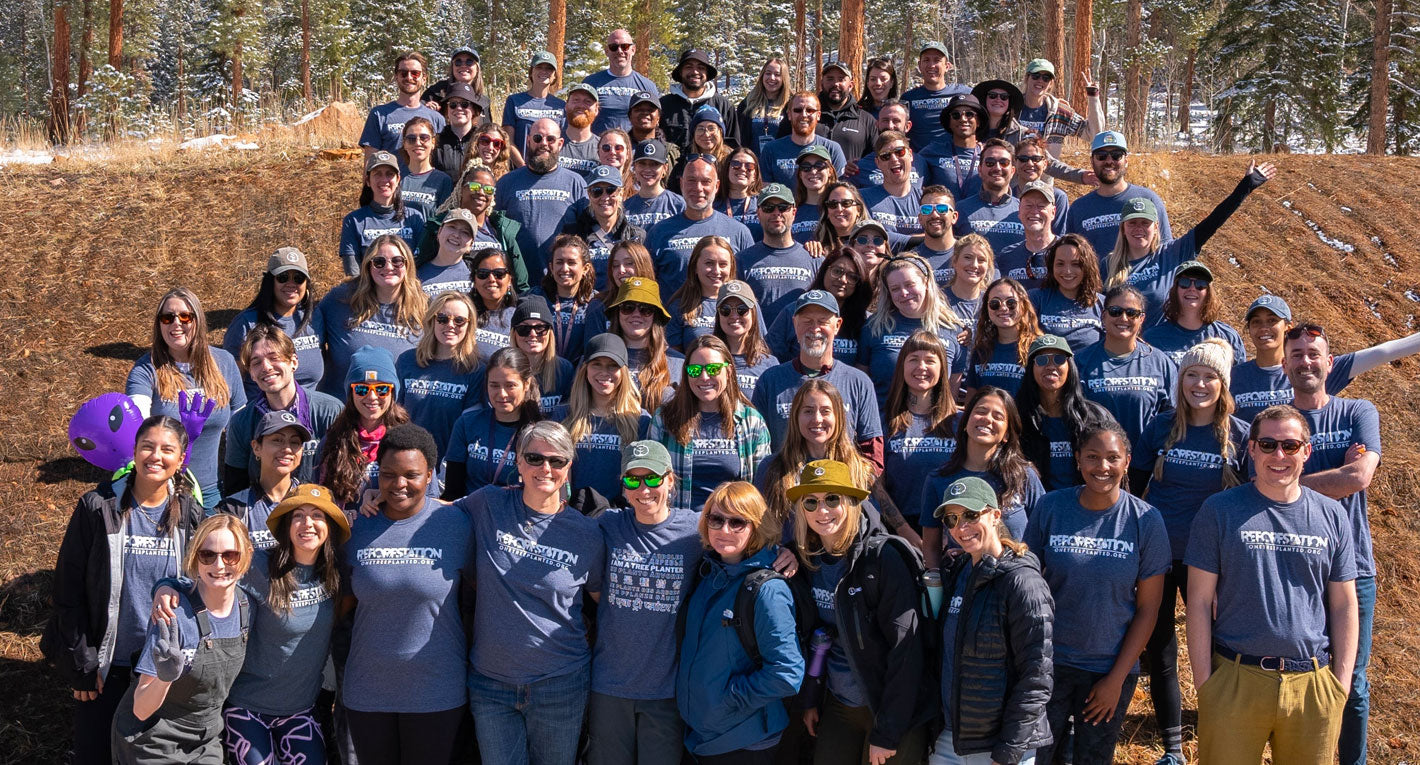The photograph captures a large group of approximately 70 people gathered on a hillside, wearing matching blue t-shirts that feature text starting with a 'P' and ending with an 'I-O-N.' Many in the group are also dressed in jackets or long-sleeved shirts, indicating a chilly, sunny day as evidenced by their sunglasses and hats. The group is arranged in several rows that climb up the hill, with everyone looking at the camera and smiling. The background is a mix of brown grass, trees, and patches of snow, suggesting a forested area. Notably, an inflatable purple alien is being held by one person on the left of the image, adding a whimsical touch to the scene.